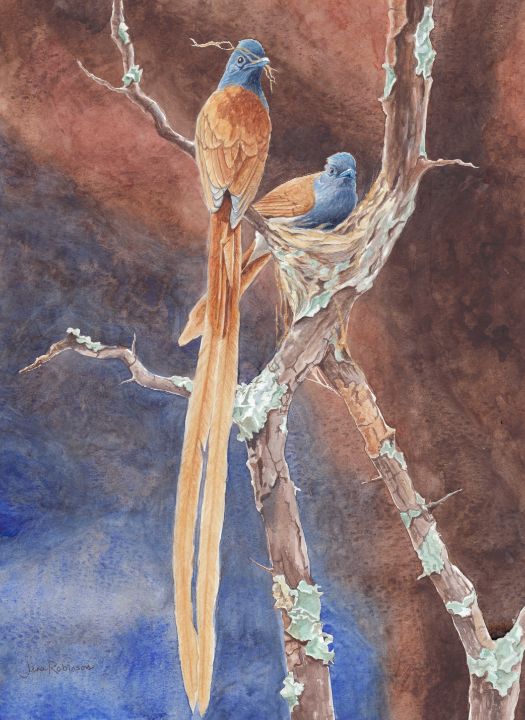This vertical rectangular painting depicts two similar-looking tropical birds sitting on the branches of a bare, dead tree. The tree's branches, devoid of any foliage, cross in the center of the scene, contributing to its stark, weathered appearance with hints of white bark and a greyish tint. The background is an abstract blend of coppery and blue tones, with a mysterious quality that suggests an out-of-focus landscape. 

The birds have blue heads, blue chests, and brown bodies, wings, and tails. Notably, the bird in the foreground has exceptionally long tail feathers that extend to the bottom of the image, while the bird behind has tail feathers about the same length as its body. Additionally, the bird in the foreground is holding nest-building material in its beak, hinting at nesting activity. Both birds appear calm and are looking off in the same direction, adding a sense of alertness to the composition. The overall color palette of the image includes hints of orange and copper, complementing the blue hues of the birds and creating a harmonious, yet stark, visual effect.